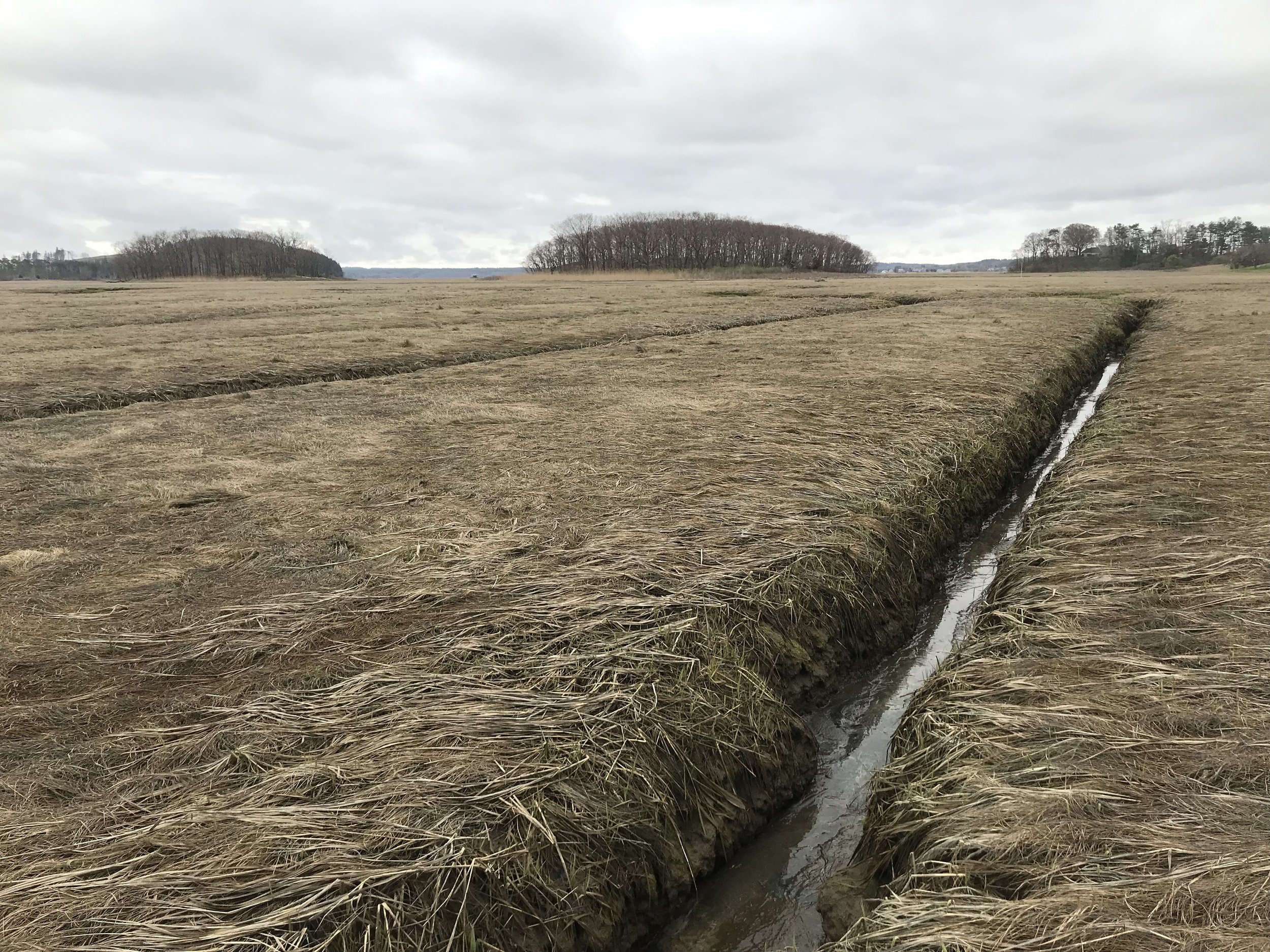This photograph depicts a barren field, likely taken in late fall or winter, with matted, dead grass or remnants of previous crops covering the ground. To the right, a small creek winds through the desolate landscape, joining a network of irrigation ditches. The sky is heavily overcast, casting a gray gloom over the scene. In the background, several clusters of mostly leafless trees stand, adding to the overall sense of dormancy and barrenness. The field is marked by a series of parallel irrigation trenches that extend into the distance, some connecting far off. The entire scene exudes a cold, dormant atmosphere, awaiting the revival of spring.